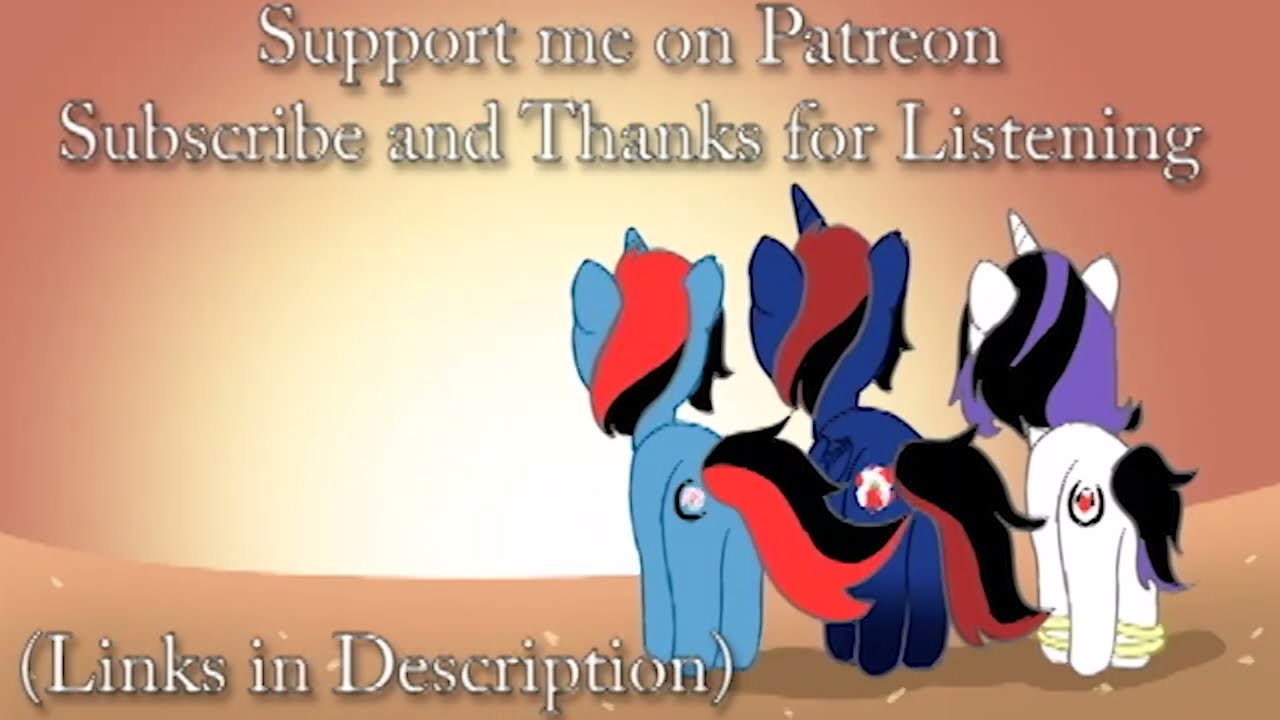The image features three My Little Pony unicorns standing on a sandy dune, predominantly on the right side of the screen, gazing towards a horizon. The horizon showcases a bright, glowing white orb at its center, radiating out into soft yellow and peach tones in the sky, gradually deepening into darker pink hues towards the edges. The dune beneath the ponies' hooves is a beige-pink color, giving the impression of a serene, otherworldly landscape.

From left to right, the first unicorn is periwinkle blue with a black and red mane and tail, adorned with a black crescent moon emblem encircling a white circle on its flank. The central unicorn is a darker bluish-purple, also with a black and red mane and tail, and features a white circle with three red spots on its hind flank. The unicorn on the far right is white, distinguished by a black and purple mane and tail, with a black "U" brand on its flank containing a red symbol with black dots within. This last pony also sports bangles around its left front and right rear hooves.

Text at the top of the image reads, "Support me on Patreon, subscribe and thanks for listening," while the lower left-hand corner includes the phrase "(links in description)." This vibrant and detailed artwork serves as a banner for Patreon support, inviting viewers with its whimsical charm and soft color palette.